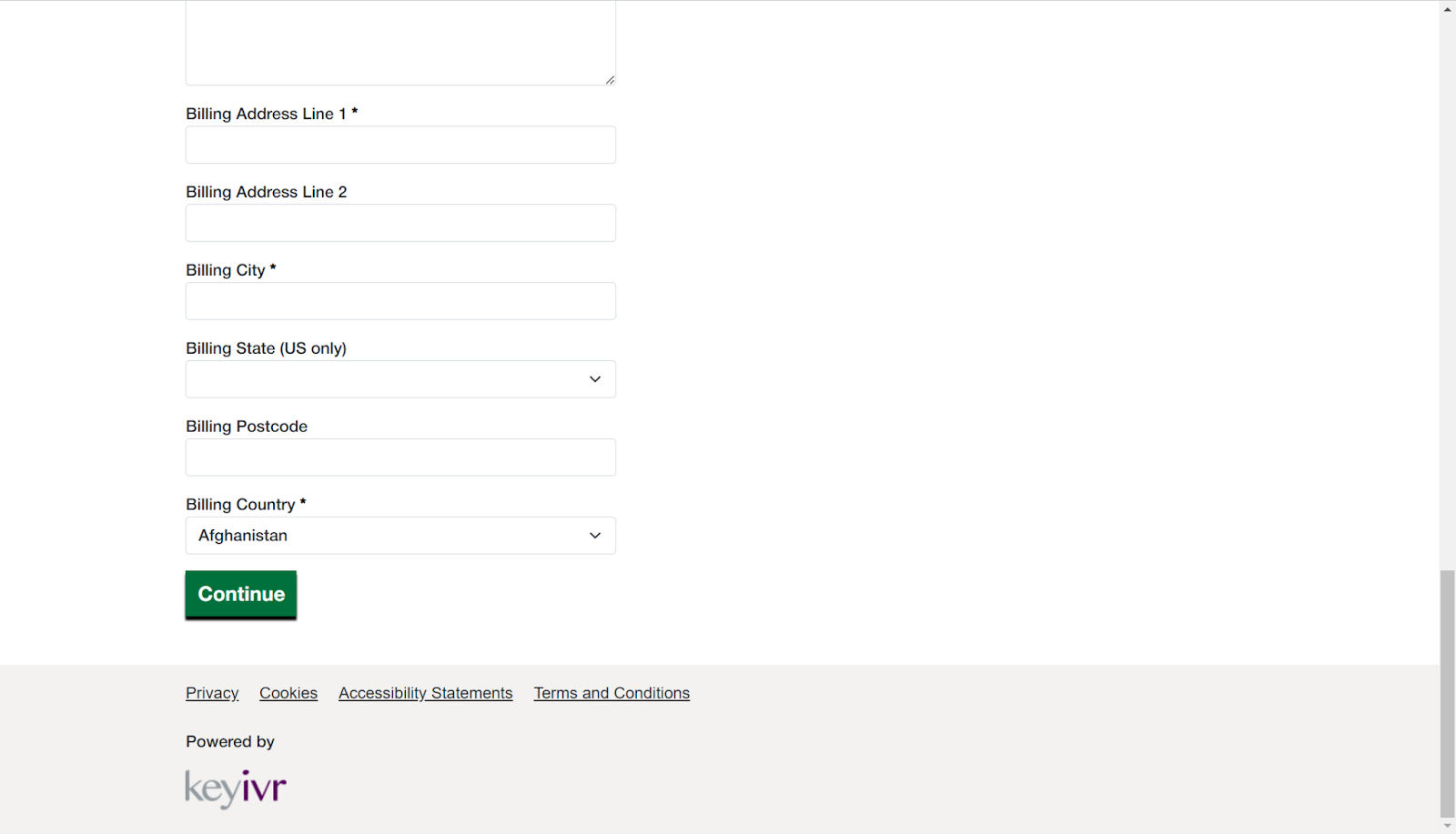This image is a partial screenshot of a web page, capturing the footer and a portion of a signup form. The top header is not visible. The background color of the main page is white, while the footer has a very light gray background. On the left side of the footer, the text "powered by" is displayed in gray letters. Below this, the company name "Key Iver" is shown, with "key" written in lowercase letters and in light gray, and "Iver" in a darker gray font. Above this area are underlined hyperlinks for privacy, cookies, accessibility statements, and terms and conditions.

The main section of the page features a signup form requesting billing information. The form fields include "Billing Address Line 1" with a corresponding light gray-traced rectangle for input. Subsequently, there are fields for "Billing Address Line 2," "Billing City," and "Billing State" (indicated as U.S. only). There is a dropdown menu for selecting the state. Further down, fields for "Billing Postcode" and "Billing Country" are available, with "Afghanistan" shown as the default option in another dropdown menu, suggesting a list of countries to choose from. At the bottom of the form, there is a green rectangle button with the word "Continue" written in white font.